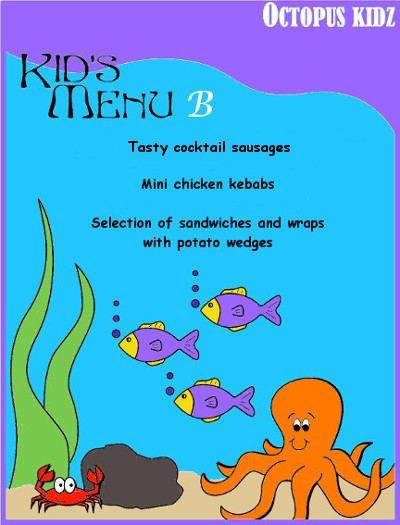The image is a vibrant, cartoonish digital illustration designed for a kid’s menu, specifically an undersea scene. Dominating the upper portions of the image, "Kids Menu B" is written in white text against a purple wavy backdrop on the left, while "Octopus Kidz" is displayed in white text on the upper right. The border of the image is a consistent purple, contrasting with the blue background that effectively conveys an underwater setting.

The menu itself lists three appealing dishes for children: tasty cocktail sausages, mini chicken kebabs, and a selection of sandwiches and wraps with potato wedges.

We also see a lively underwater scene depicted below this list. Swimming amongst the blue waters are three purple fish with yellow faces and fins, blowing bubbles as they face left. Nearby, an orange octopus spreads its tentacles, and a playful red crab with expressive eyes peeks out from behind a brown rock. Green underwater plants add a natural touch to the setting, enhancing the enchanting, undersea atmosphere of the illustration.